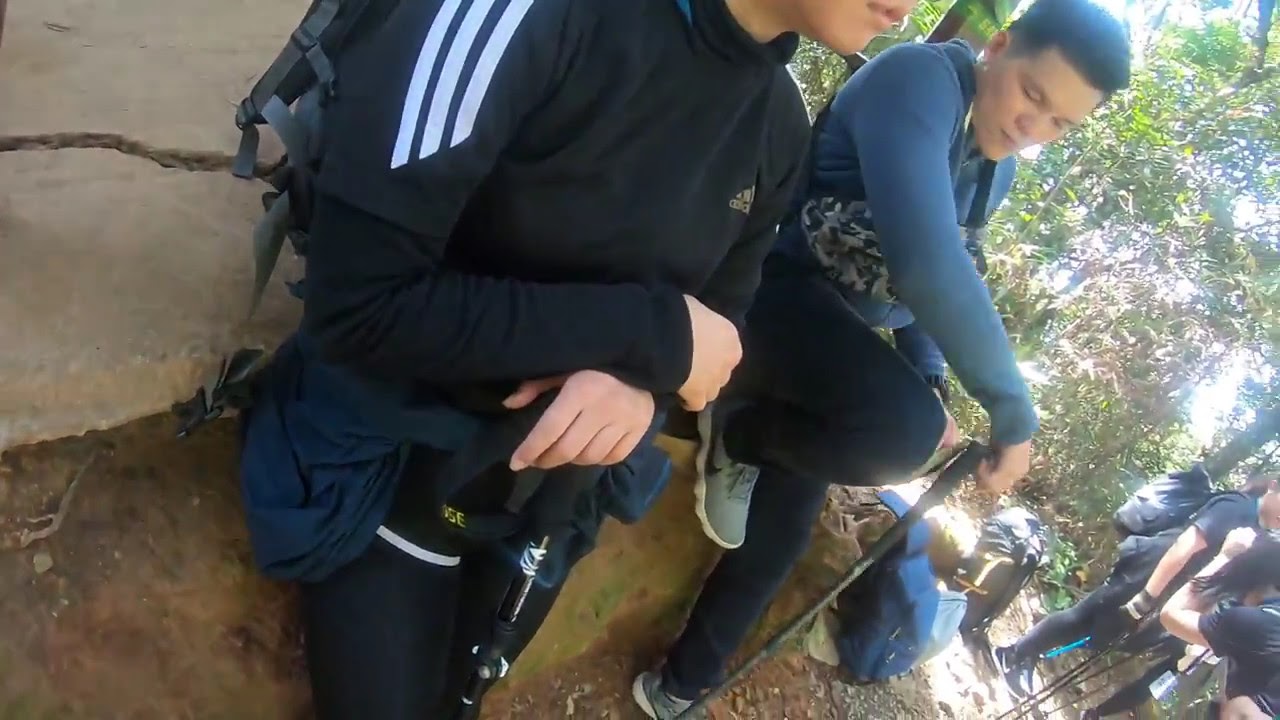The photograph captures an outdoor scene of a hiking group taking a rest. Central to the image are two individuals, a man and a woman, both seated on a rock amidst a forested trail. The woman, identifiable by her black Adidas long-sleeve shirt with white stripes and black pants, has a backpack. The man, next to her, is dressed in a blue long-sleeve shirt, black pants, and blue and white shoes, and he holds a hiking stick. The background reveals several other hikers, also equipped with backpacks, wearing predominantly black, and the area is dappled with sunlight filtering through the trees. The trail itself is rough, covered in dirt, rocks, and pebbles, indicating a rugged daytime hike.